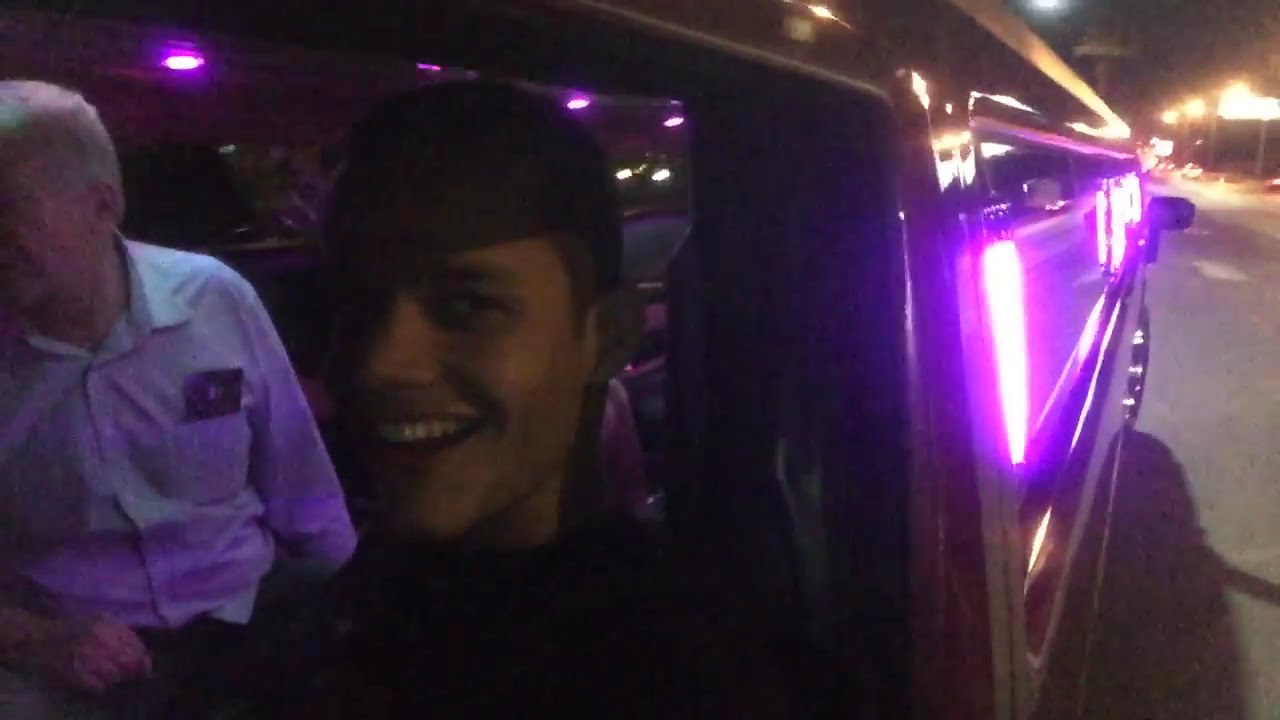The image captures a detailed and lively scene inside and around a stretch limousine. On the left half of the picture, there are two people visible. Closest to the edge, an older man with gray hair, wearing a long-sleeved collared shirt, has something in his left breast pocket. His left ear and a side profile of his face are visible as he seems to be engaging with someone off-frame. Beside him, a younger man is clearly captured smiling, possibly taking a selfie with his smartphone. Pink LED lights ornament the exterior windows of the limousine, casting a vivid glow that bathes both the inside and outside of the vehicle. The scene is illuminated further by streetlights visible in the upper right corner of the image, suggesting they are on a city street. The limo, evidently a long stretch vehicle, showcases wheels with a side mirror above, contributing to the overall grandeur of the setting. Both individuals appear to be enjoying themselves, adding a cheerful ambiance to this vividly lit scene.